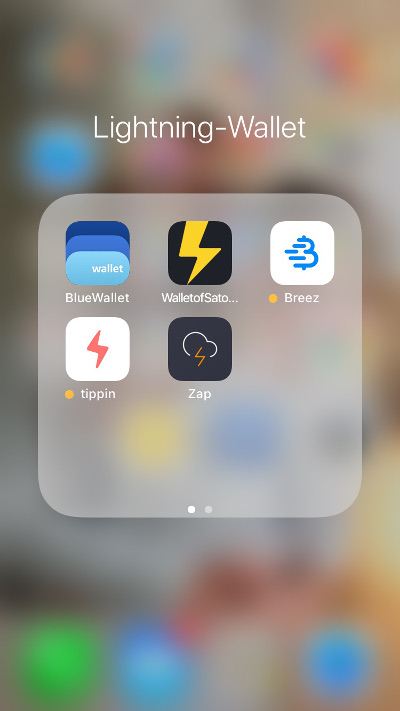This screenshot, taken from an iPhone, captures a blurred background with central, bold, white text that reads "Lightning Dash Wallet." Below this, in a light gray square, are multiple app icons arranged in two rows.

**Top Row:**
1. **First Icon**: A dark blue square, followed by a mid blue square, and a light blue square with rounded corners, creating an almost oval shape. This light blue square, closer to cyan, features white text on the right that reads "Wallet" with "Blue Wallet" underneath, identifying the app.
2. **Second Icon**: A black square with rounded corners displaying a yellow lightning bolt, labeled "Wallet of STO..." due to truncated text.
3. **Third Icon**: A blue square with a white 'V' resembling the Bitcoin 'B' with three horizontal lines, encircled by yellow. To the right, it is labeled "VREEZ," with a capital 'V' and the rest of the letters in title case.

**Bottom Row:**
1. **First Icon**: A white square with rounded corners featuring a red lightning bolt within an orange circle. White text beside it reads "tipping," with a lowercase 't.'
2. **Second Icon**: An off-black square with a partially drawn cloud silhouette and an orange lightning bolt emerging from the incomplete area. Underneath, it is labeled "ZAP" with a capital 'Z'.

At the bottom of the square, there are two navigation circles. The left circle is white, indicating the current page of apps, while the right one is gray, suggesting the presence of another app page.